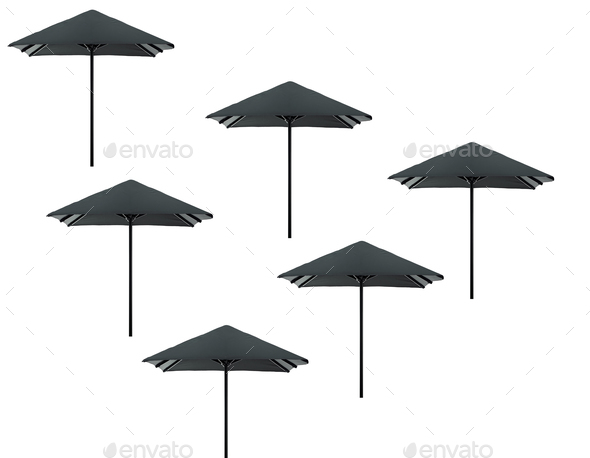The image features six black umbrellas, each with a distinctive design featuring dotted lines forming an X pattern across them. These umbrellas are arranged against a white background in a triangular formation pointing towards the left corner. Specifically, there is one umbrella in the top left corner, two directly below it to the right, and three more beneath them, also diagonally aligned to the right. Visible throughout the image is a light gray watermark with the text "Envato," indicating that it is a stock photo. Each umbrella has a long black handle, contributing to the cohesive visual theme. The repeated and scattered "Envato" watermark further emphasizes the image's stock photo nature.